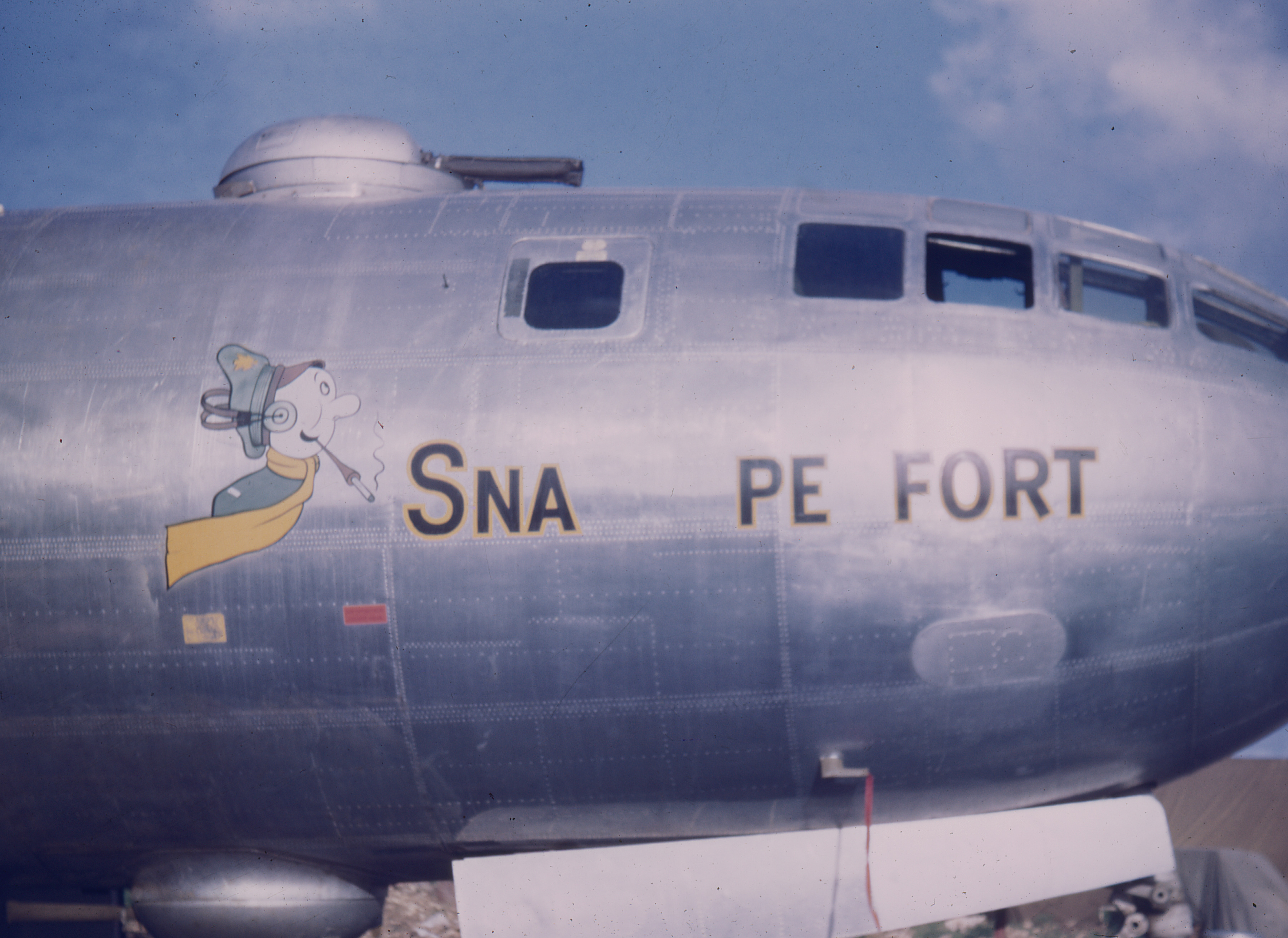The image captures a nostalgic scene featuring the front portion of a vintage silver airplane or blimp, seemingly grounded on a dirt surface under a blue sky dotted with soft white clouds. The image, characterized by its low resolution and faded appearance, highlights the aircraft's horizontal orientation as it faces right. Distinctive features include a tank-like structure atop the plane, possibly a weapon. Across the metallic surface of the aircraft, the text "SNA PE FORT" is prominently displayed in black letters with a yellow outline. Adjacent to the text is a vividly detailed cartoon character that resembles a pilot, sporting a yellow scarf, a green uniform with a matching hat, and a headset. The character's face bears a whimsical resemblance to a dwarf from Snow White, complete with a long pipe emitting smoke. Four windows line the side of the plane, adding to the antique aviation charm of the scene.